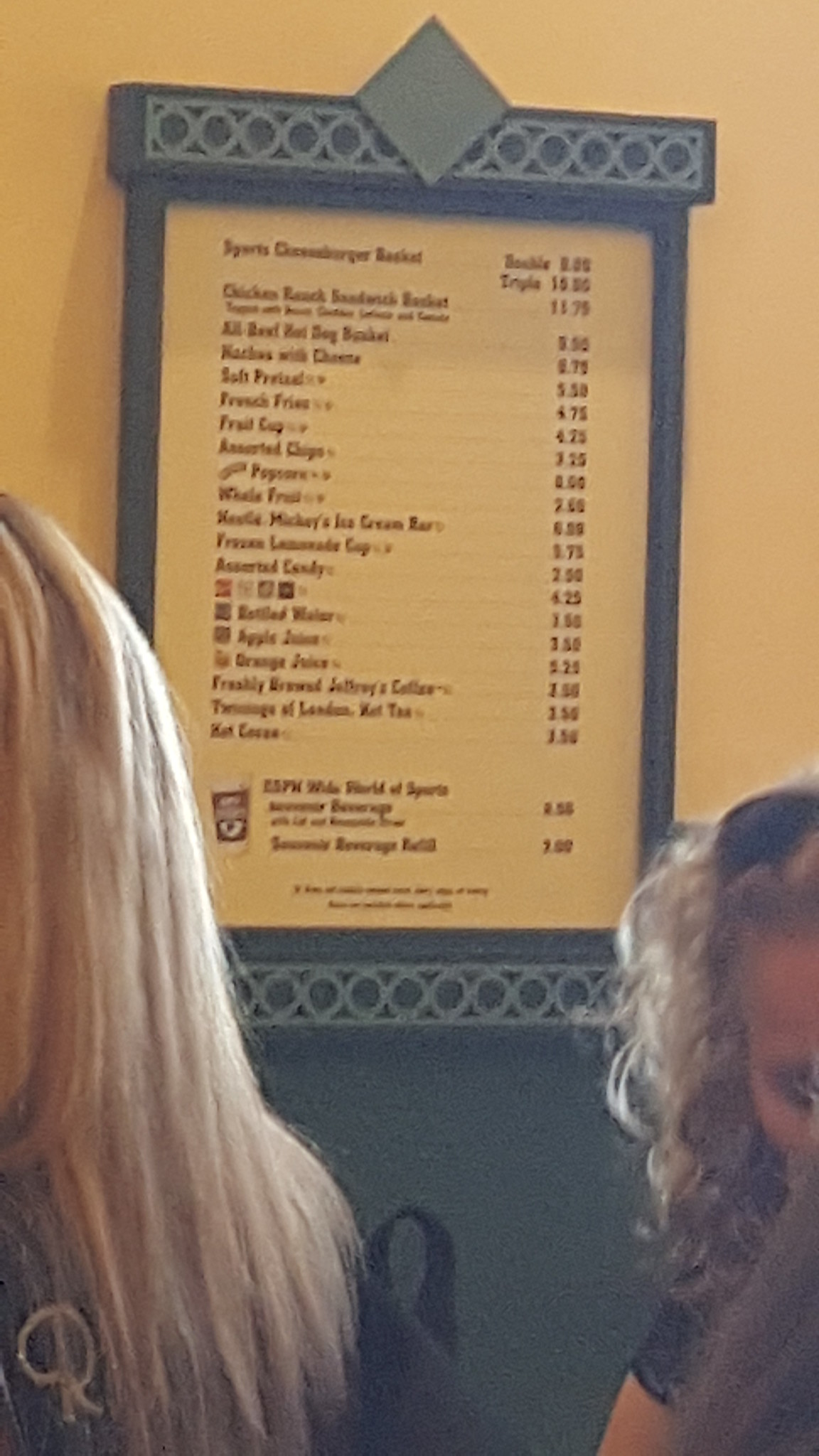This photograph, though slightly out of focus, captures a cozy moment in a restaurant characterized by its warm and inviting decor. Taking center stage in the background is a menu board, suspended from a bluish-gray and yellow wall. The menu itself features a yellow background framed by a bluish-gray border adorned with a series of lighter gray circles; its contents are blurred but reveal items like Mickey's ice cream bar, frozen lemonade cup, salted pretzel, french fries, and assorted chips. A distinctive gray diamond shapes sits atop the center of the menu board.

In the foreground, two women are conversing. The woman on the left is seen from behind, her long, straight blonde hair cascading past her shoulders. She wears a garment with the cursive letter "R" visible on the lower left side, and a black strap can be discerned over her shoulder. The woman on the right, partially visible, sports curly blonde hair. She has fair skin and what appears to be either a black headband or dark sunglasses resting atop her head. A glimpse of her dark eye is visible, beneath which she wears a dark, short-sleeved upper garment. This candid scene beautifully captures a moment of everyday life against the backdrop of a charming restaurant setting.